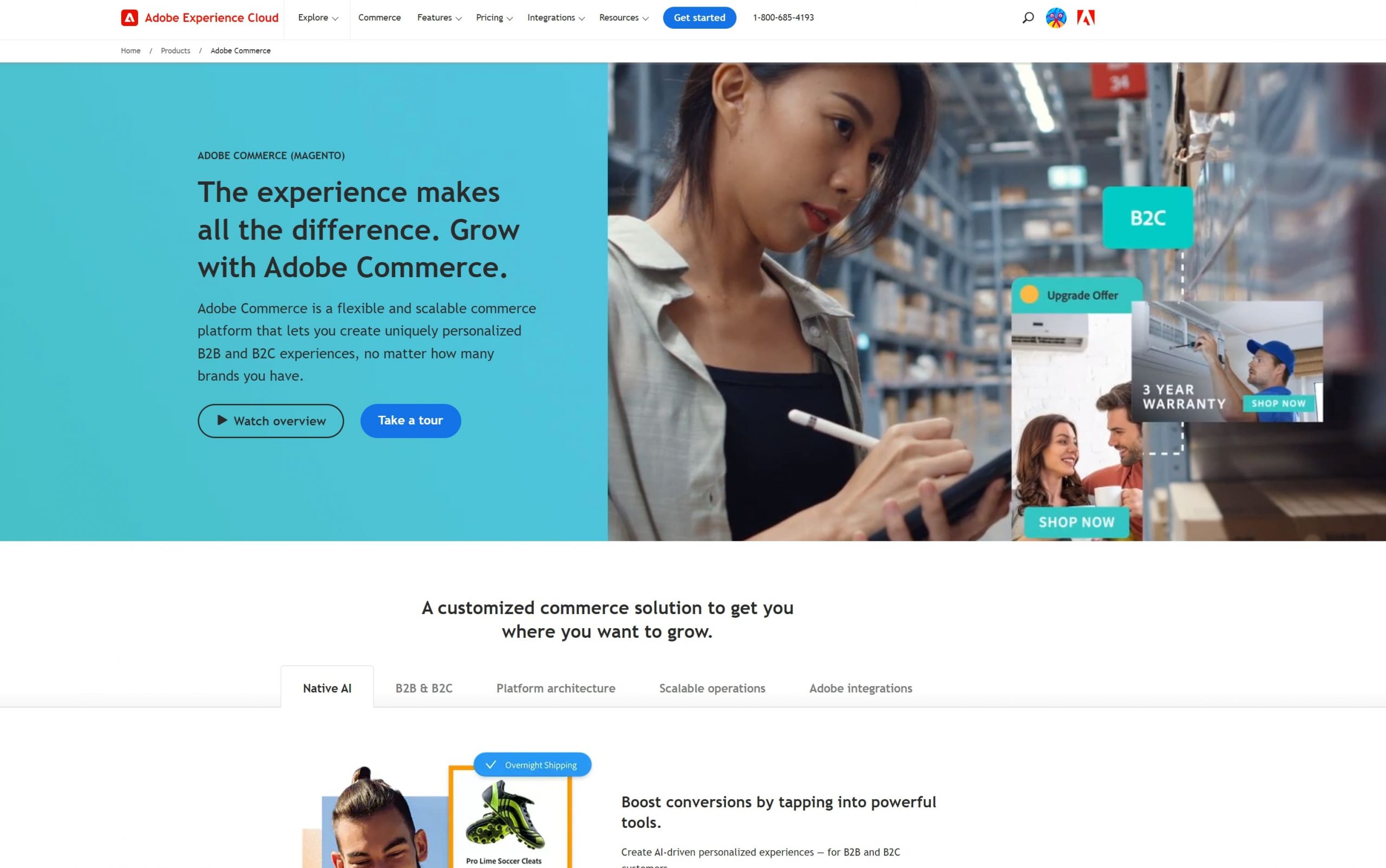The image is a screenshot of a website showcasing Adobe Experience Cloud. In the top left-hand corner, there is the Adobe Experience Cloud logo and text in red font. Dominating the page below is a large image of a woman writing with a white stylus on a tablet or cell phone. The woman is looking downward and appears to be working in a warehouse setting.

To the left of the image is the title and description: "The experience makes all the difference. Grow with Adobe Commerce. Adobe Commerce is a flexible and scalable commerce platform that lets you create uniquely personalized B2B and B2C experiences no matter how many brands you have."

Below the description are two buttons: one on the left labeled "Watch Overview" and the other on the right labeled "Take a Tour." The bottom left and bottom right corners feature open, white spaces, and the overall background color of the website is white.